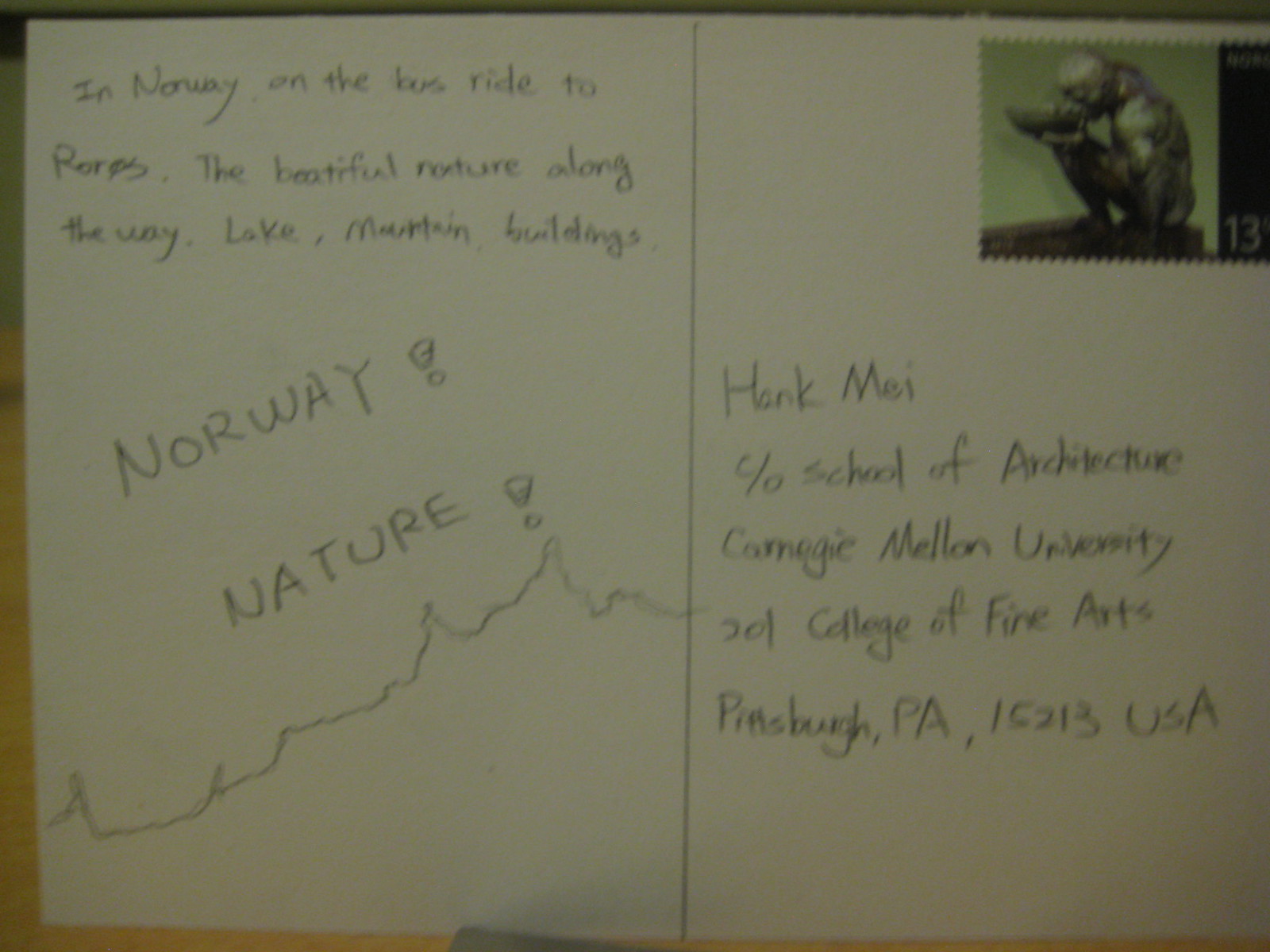This blurry, dark photograph or scan captures the back of a postcard. In the upper left corner, handwritten text reads, "In Norway, on the bus ride to [unintelligible], the beautiful nature along the way: lake, mountain, buildings." The postcard also includes the phrases "Norway nature" and features a small sketch resembling an altitude or elevation graph, possibly indicating a map or a road path. The recipient is Hank May, care of the School of Architecture at Carnegie Mellon University, 201 College of Fine Arts, Pittsburgh, PA 15213, USA. In the upper right corner, there's a dark green stamp with the number 13 on it, although it does not appear to have a postmark, raising questions about whether the postcard was ever sent or delivered.